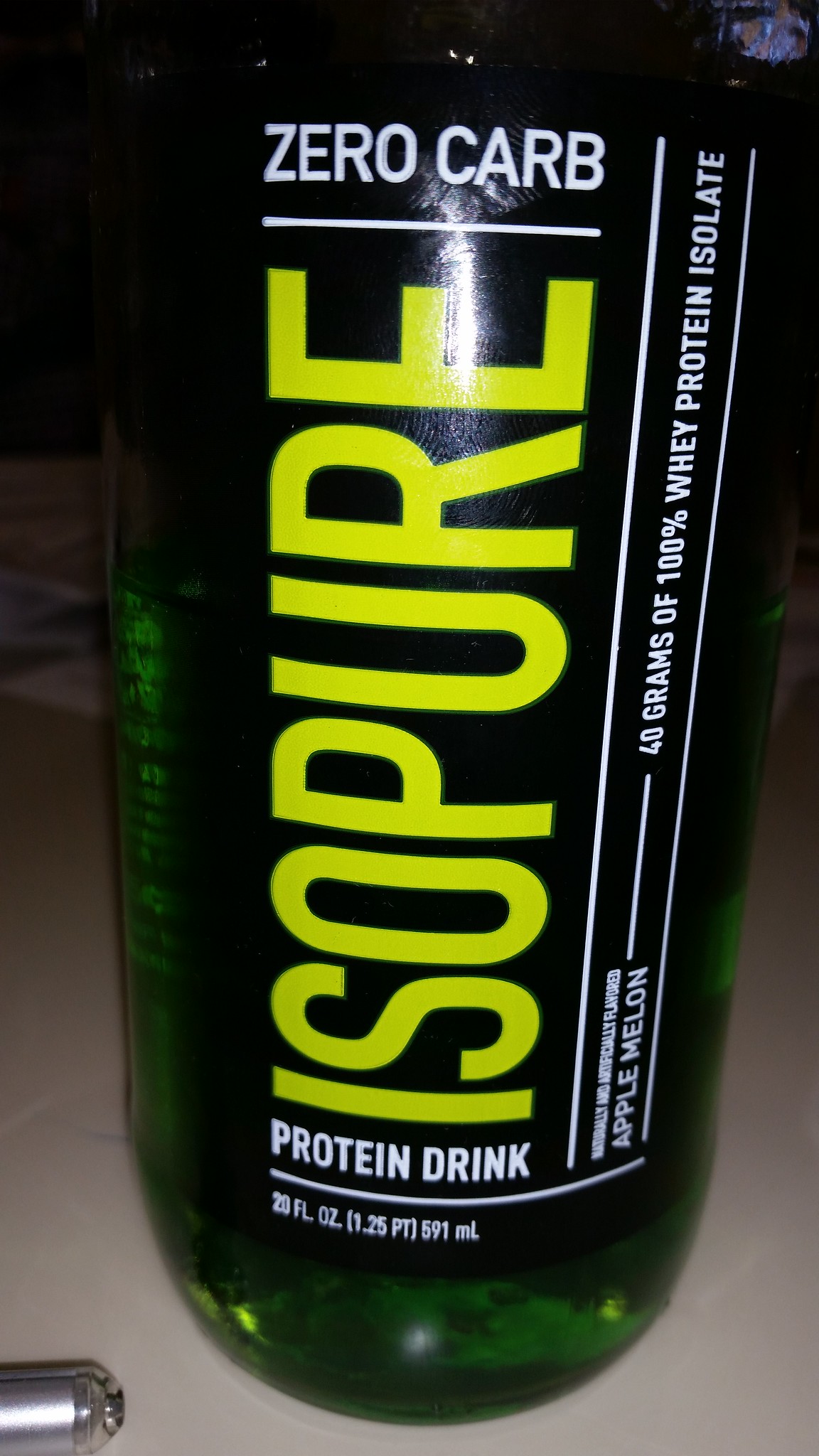This vertical close-up photograph captures a black can with bright yellow and white text, positioned on a beige counter. The can prominently displays the brand name "Isopure" in vertical text that runs from bottom to top, requiring the viewer to tilt their head to read it. Below the brand name, the text includes details of the contents: "Protein Drink, 20 Fluid Ounces, 1.25 Pint, 591 ml." Adjacent to this, additional white text provides further information: "Apple Melon, Naturally and Artificially Flavored, 40 Grams of 100% Whey Protein Isolate." Across the top of the can, the text "Zero Carb" stands out, highlighting a key nutritional attribute of the drink. The design of the can is visually striking, combining bold typography with a minimalist color palette on the textured surface of the counter.